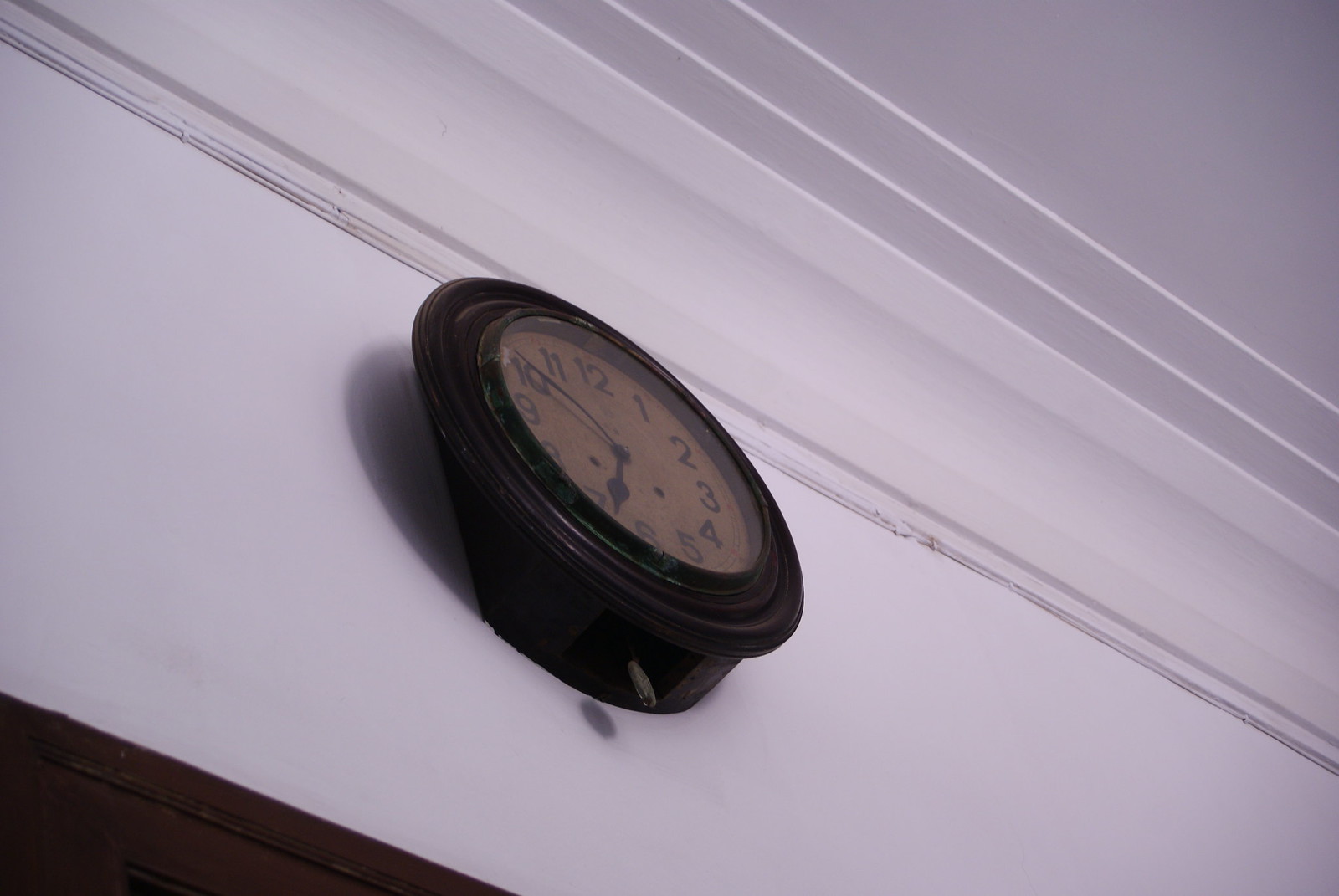This photograph captures a striking view from below of an old-fashioned wall clock mounted high near the ceiling. The setting features a white wall and ceiling, with some intricate architectural details. Just above the clock, there's an ornate, wide, thick molding that adds a dramatic flair, and further up, the ceiling showcases diagonally placed wooden strips creating an additional decorative element. The clock itself is encased in a dark mahogany or dark walnut wooden frame, lending it a classic appearance. The clock's faded tan face displays vintage-style numbers, and the time reads ten minutes before seven o'clock, as indicated by the black hands. In the lower right corner of the image, part of a dark brown door frame is visible, grounding the otherwise airy composition. Overall, the photograph combines elements of timeless elegance with subtle architectural intricacies.